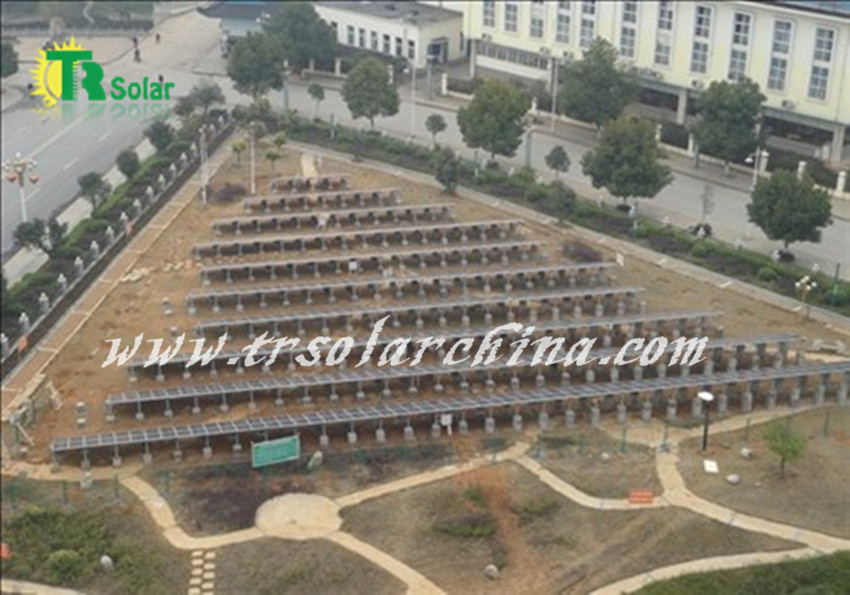The aerial photograph showcases a large, triangular field within a city, dominated by numerous rows of solar panels, likely totaling over a hundred. The solar panels are arranged in graduated rows which widen towards the bottom of the image, emphasizing the triangular shape of the area. Surrounding the solar panels are brown pavements and scattered trees, bushes, and plants that add a touch of greenery to the scene. Beyond the solar array, there's evidence of a public park with walkways, benches, and scattered people, suggesting it's a recreational space as well. The background reveals roads, buildings, and some pedestrians, framing the triangular field within an urban environment. Two watermarks are visible: one in the top right corner stating "TR Solar" with a green inscription and a yellow sun icon, and another across the front reading "www.TRSolarChina.com" in white text. Additionally, in the top right corner stands a yellow and grey building. This suggests that the field is part of a solar power initiative in China, potentially advertised by TR Solar.